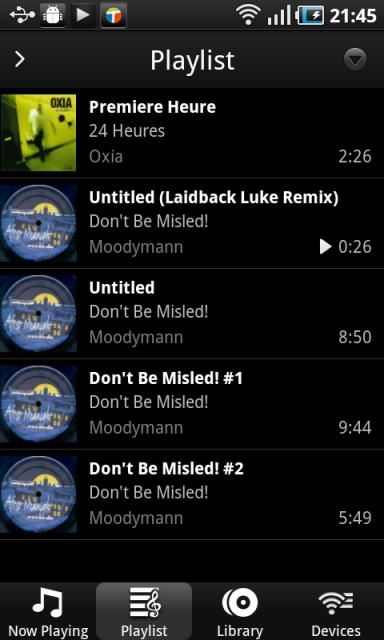### Detailed Caption

The image showcases a cell phone screen displaying a playlist interface with a black background. At the top, in the largest white text on the page, the word "Playlist" is prominently featured. On the left side of the screen is a vertical column displaying album covers beside the track titles and their respective playtimes.

Below the "Playlist" heading, the first entry features a square image that is slightly out of focus. In the upper right corner of this image, the text "OXIA" is visible. The image depicts a person and includes French text that reads "Premier Heureux, 24 Heures Auxiles, 2:26."

The next entry down features a blurry cover image that is difficult to decipher but appears to include a circular design, a possible airplane, and a city silhouette. The associated text reads "Untitled, Laidback Luke Remix, Don't Be Misled, Moody Man" with a playtime of "0:26."

Following this, the third blurry cover image repeats the circular pattern. The accompanying text is "Untitled, Don't Be Misled, Moody Man" with a playtime of "8:50."

The fourth entry again showcases a circular blurry cover image, labeled "Don't Be Misled, Number 1, Don't Be Misled, Moody Man" and lists its duration as "9:44."

The final image mirrors the previous three with the same blurred circular design. It is labeled "Don't Be Misled, Number 2, Don't Be Misled, Moody Man" with a playtime of "5:49."

Along the bottom of the screen, there are navigation options including "Now Playing," which is highlighted, alongside "Playlists," "Library," and "Devices."